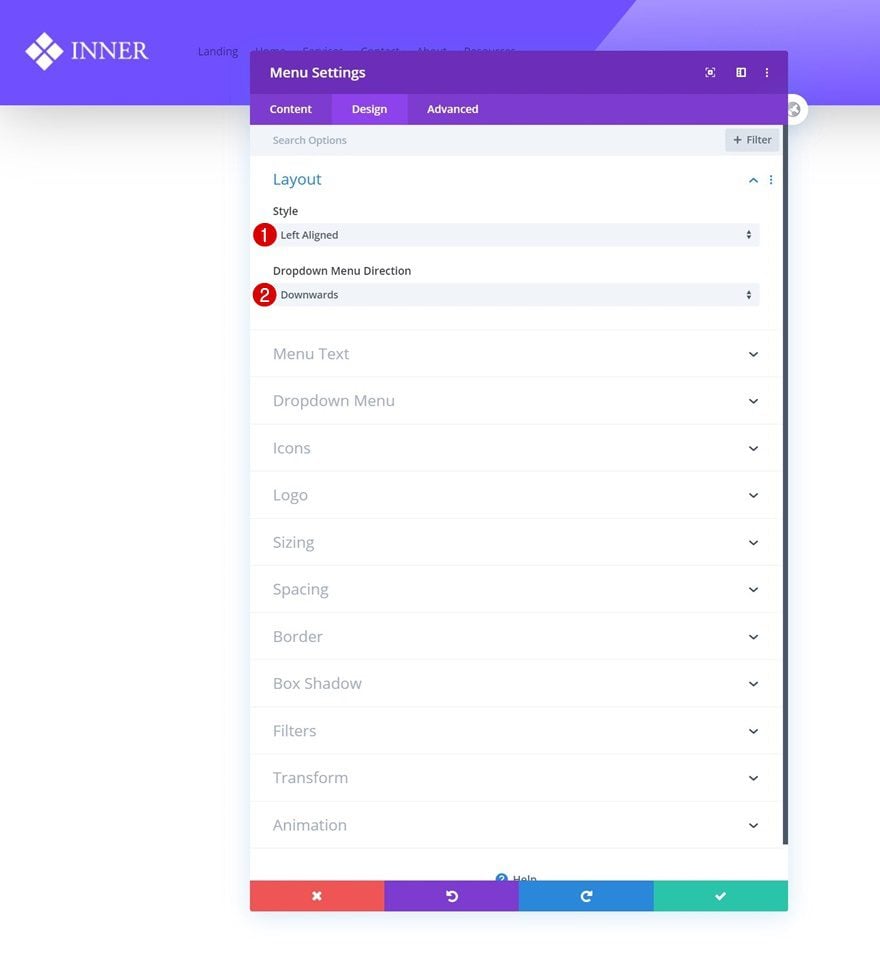The image depicts a website interface with multiple layers of menus. At the top, there is a purple banner with a gradient effect, transitioning from a darker shade on the left to a lighter, more faded purple on the right. On the left side of this banner, there is a small diamond icon followed by the word "inner" in white text. This portion is slightly obscured by a secondary, darker purple menu bar that has popped open on top of it.

The darker purple menu bar displays the text "Menu Settings" in white and includes three main options: "Content," "Design," and "Advanced." Below this, a drop-down menu with a white background presents additional options for customization. Among these, "Layout Style" is prominently featured with a white number "1" inside a red circle, indicating its current selection on left alignment. Another option, "Drop-Down Menu Directions," has a digit "2" in the same red circle next to the word "Downwards," suggesting ongoing adjustments.

The remaining options in the drop-down menu are in grayscale and appear less emphasized, almost as though they are secondary or currently inactive. Each of these options can be clicked to modify various settings according to user preferences.